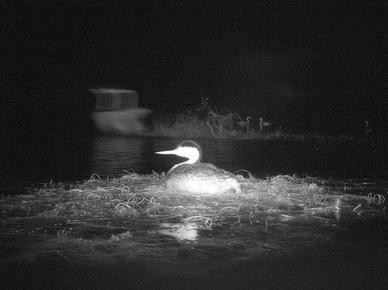In a grainy black and white nighttime photograph, a duck-like bird with a lighter beak and head is partially illuminated by a strong light source while it rests on a cluster of grass and weeds floating on a body of water, possibly a lake or stream. The scene is shrouded in almost total darkness, with only faint, blurred outlines of distant grass patches and a possible boat barely visible in the background. The bird appears to be nesting on what looks like a small, vegetative island within the water, adding to the enigmatic and serene atmosphere captured in the image.